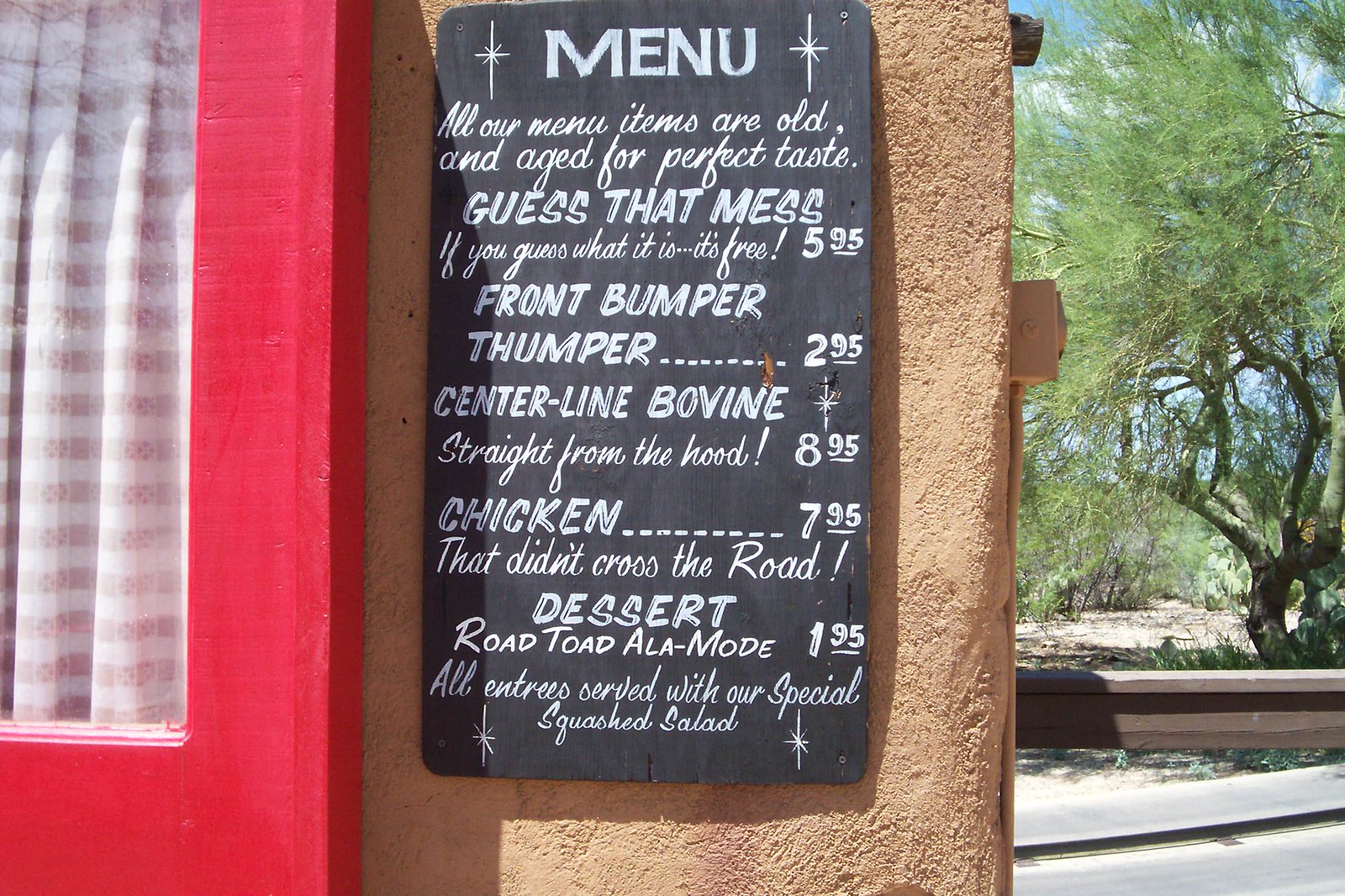The photograph captures an outdoor scene featuring a quirky menu displayed on the side of a clay-colored stone building. On the left side of the image, the back of a red and white striped curtain hangs almost the length of the building. This curtain is framed by thick red wood. Adjacent to it, there is a rectangular blackboard with a chalkboard appearance, prominently showing the menu in white text. 

In the upper left corner of the chalkboard, a plus sign with a star in the middle is drawn. "MENU" is boldly written in all caps, flanked by the same star-cross symbol to the right. The menu humorously claims "ALL OUR MENU ITEMS ARE OLD" and "AGED FOR PERFECT TASTE." Listed items include:

1. "GUESS THAT MESS" – Guess the dish correctly for it to be free, otherwise priced at $5.95.
2. "FRONT BUMPER" – $2.95, aligned with "THUMPER."
3. "CENTERLINE BOVINE" – Price not specified.
4. "STRAIGHT FROM THE HOOD!" – Cursive, $8.95.
5. "CHICKEN" – $7.95, followed by the phrase "THAT DIDN'T CROSS THE ROAD!"
6. Under a centered heading "DESSERT":
   - "ROAD A LA MODE" – $1.95.
   - In cursive, "ALL ENTREES SERVED WITH OUR SPECIAL SQUASHED SALAD."

To the right edge of the photo, a tree with green leaves stands against a backdrop of blue sky and white clouds. A low brown wall runs in front of the tree, and the bottom right corner reveals gray concrete pavement.